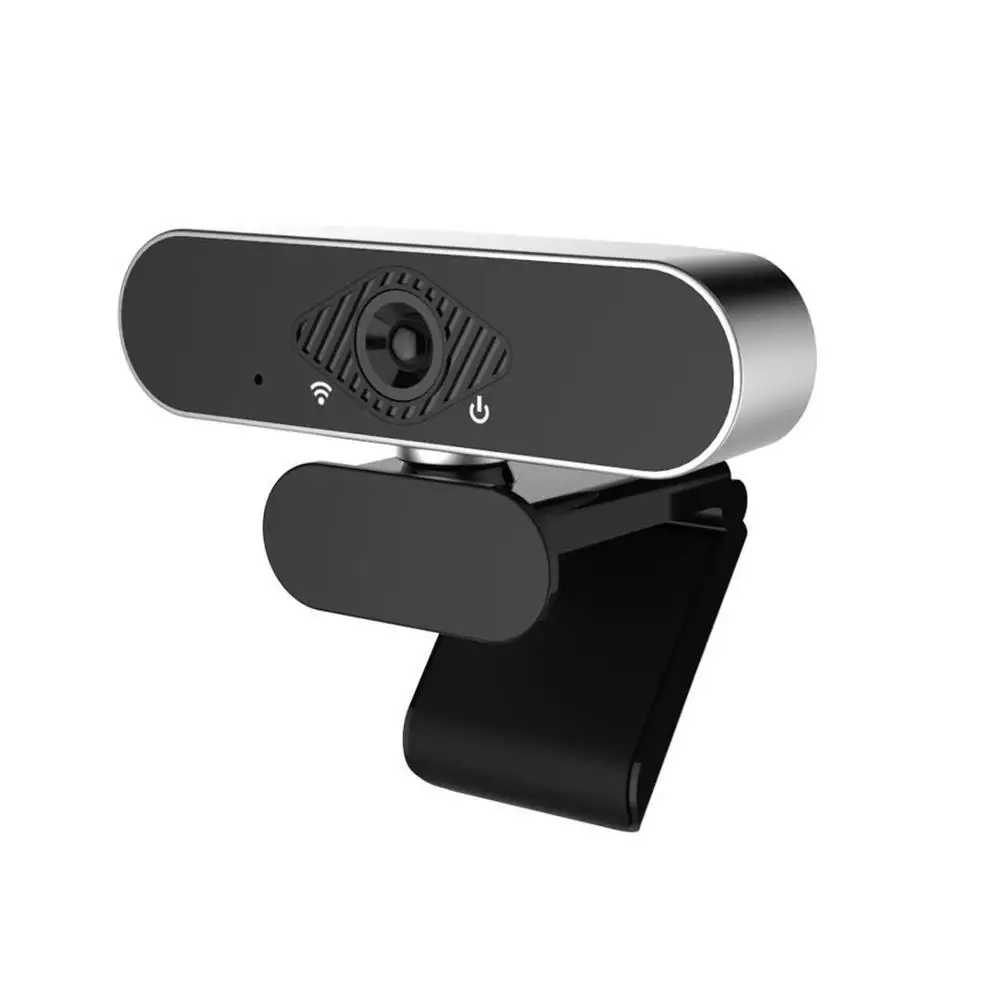The image features a sleek, modern webcam prominently displayed against a plain white background. The main body of the webcam is constructed from shades of grey and black plastic, with a shiny grey encasement surrounding a more matte front surface. The overall shape of the webcam resembles an open band-aid or a stylized eye, with a black face at the front. Central to the front face is a flush-mounted lens, surrounded by a small hole on the left side likely serving as the microphone or an LED indicator. Additionally, the webcam includes symbolic indicators with a white Wi-Fi logo and a power button on the right and left sides, respectively, suggesting both are currently inactive. The upper part of the webcam also features a textured section, possibly for additional button controls. The device sits atop a cylindrical, folded base, designed to clamp securely onto a monitor. The polished silver outline and the contrast of grey and black give the webcam a refined, professional appearance suitable for desktop setups.